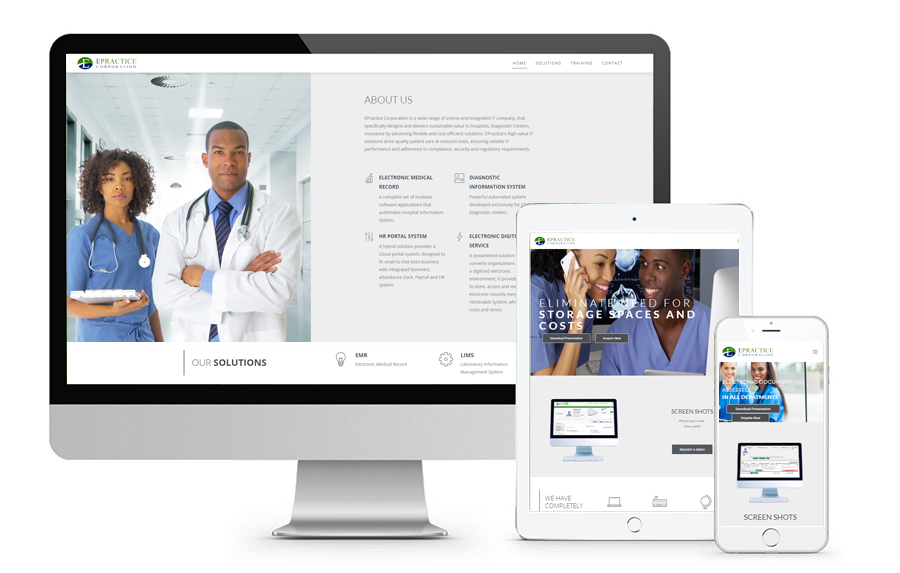The image depicts a multi-device workspace setup, showcasing a laptop, a tablet, and a smartphone. The laptop is positioned centrally with its screen slightly shifted to the left, featuring a distinctive design. The screen is framed with a black border on the left and along the bottom, while the top and right side are edged in gray. Encased within is a white background displaying a green and blue circular logo with the letter 'E', followed by the text "ePractice" in green. Below this header, though indistinct, there are some text elements. The right section of the laptop screen features clickable black text options labeled "Contact", "Training", "Solutions", and "Home". 

Depicted on the left side of the laptop screen is an image of a female nurse, characterized by her shoulder-length hair, dressed in blue scrubs, holding a chart, and wearing a stethoscope. Standing next to her is an African American doctor, notably taller, attired in a white coat, blue shirt, and blue tie, also with a stethoscope, arms crossed in a confident pose. To the right, a section labeled "About Us" appears, accompanied by smaller, harder-to-read text.

The tablet, partially overlapping the lower right corner of the laptop, presents a split-screen image. The left side shows a woman conversing on the phone, dressed in scrubs and smiling. The right side features a man in scrubs, also smiling and seemingly engaged with the woman. Additional text is present around this imagery, albeit small and not easily readable.

In the bottom right, a smartphone overlaps the tablet, depicting two individuals outdoors. Dressed in blue scrubs, they both face the camera, smiling warmly. Surrounding this image is further text, consistent with the other devices, characterized by its small and detailed nature.